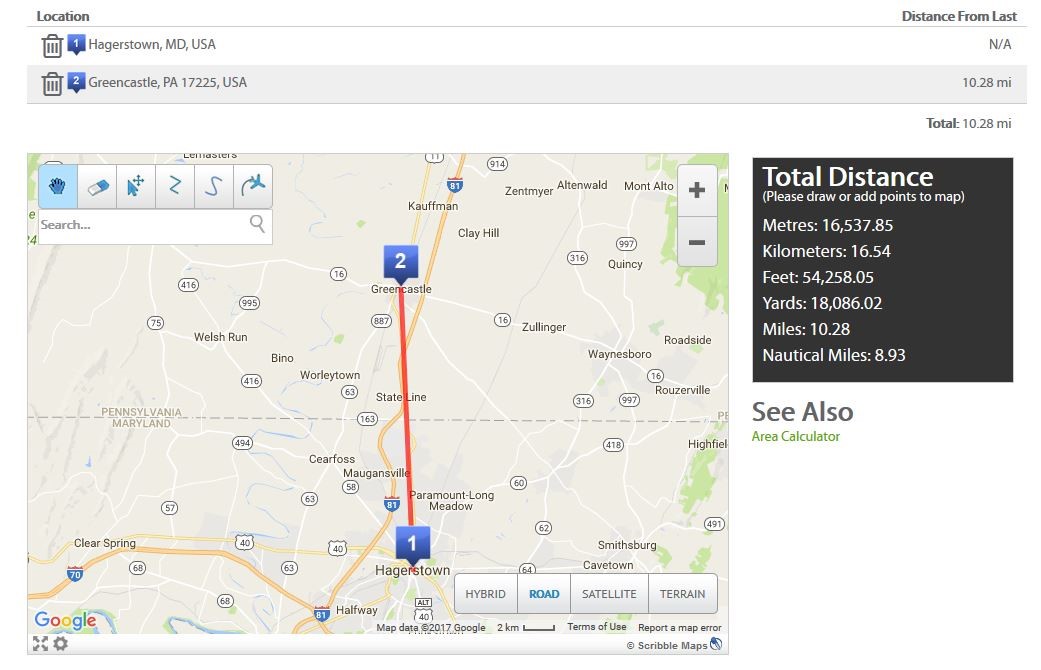The image displays a detailed route map between Hagerstown, Maryland, and Greencastle, Pennsylvania. At the top, the word "location" is highlighted, with a trash can icon next to it, indicating the option to delete it if needed. The map specifies the distance from the starting point, Hagerstown, MD, to the destination, Greencastle, PA, which is precisely 10.28 miles. The map, positioned towards the bottom, shows Hagerstown in the south, marked with a blue box labeled '1'. A red line indicates the direct path to Greencastle.

The map offers various viewing options including hybrid, road, satellite, and terrain. Currently, the view is set to road, displaying all streets, side streets, and interstates. In the top right corner of the map are plus and minus icons for zooming in and out.

To the right of the map is a black box with white text that details the total distance in various units: approximately 16,000 meters, 16.5 kilometers, 54,000 feet, 18,000 yards, 10.28 miles, and 8.93 nautical miles. Below this information is a grade C notation and an area calculator for further configurations. The map also features a search bar at the top and six additional tools above it for more detailed map functionalities.